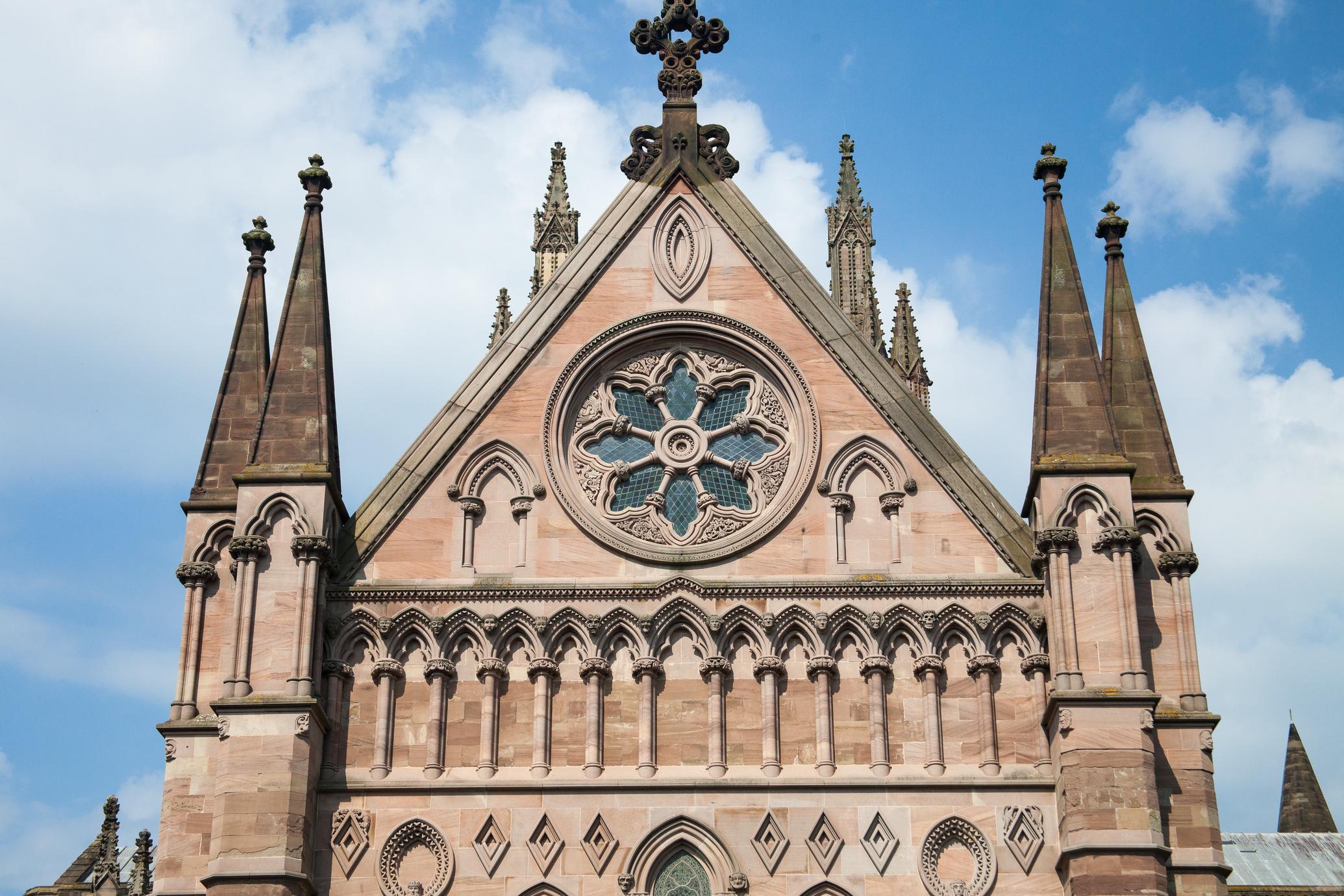This detailed photograph captures the upper portion of a magnificent, ancient church, believed to be from the medieval era. The structure is primarily built from a pinkish-brown stone, giving it an aged, majestic appearance. Prominent in the image are several turret-like spires, with four clearly visible at the front and more peeking from behind. The steeply pointed gable roof is adorned with an ornate cross at the very apex, which features intricate frilly decorations at its four points.

Central to the facade is a large, round window, designed in a wheel-like pattern that resembles stained glass. Flanking this prominent window are two smaller arched openings. Beneath this section, the facade is enriched with elaborate scrollwork, featuring numerous columns and pointed arches. The lower part of the visible structure exhibits a series of arches and diamond-shaped decorations. This intricate blend of architectural elements, coupled with the overall grandeur, points to possible Byzantine influences. The photo offers a detailed view of the upper facade, captured from a slightly elevated point, emphasizing the elaborate details against a backdrop of clear sky.